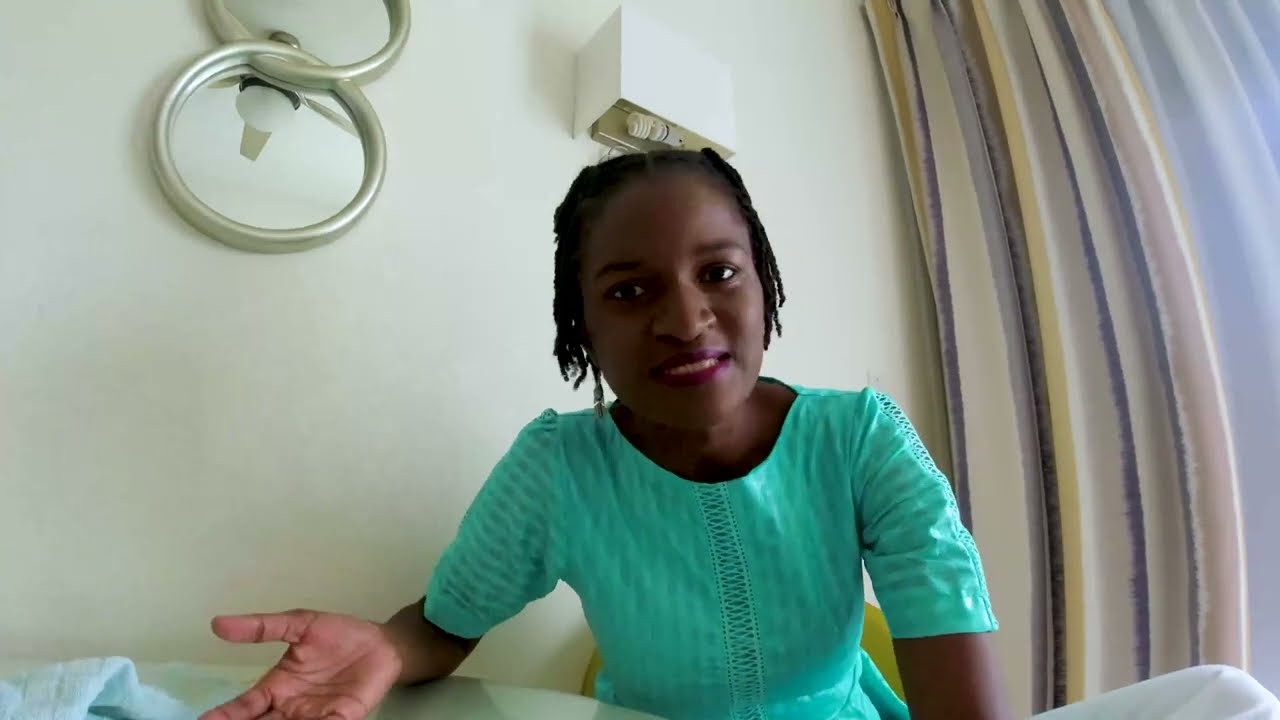The image captures a young African woman, likely in her early 30s, during a video chat. She has intricate thin braids in her black hair and is dressed in a turquoise or aqua dress with darker green vertical stripes. The woman is seated at a round table, leaning her right elbow on it with her open palm facing up as she speaks to the camera. Behind her is a white wall adorned with a white sconce and a silver metal sculpture resembling intertwined rings. To the right of the sculpture is a very tall window draped with long tan-colored curtains, allowing some natural light in. The lower part of the image also reveals her white pants and a blue rag placed next to her hand. She appears to be wearing red lipstick, adding a touch of color to her poised look.